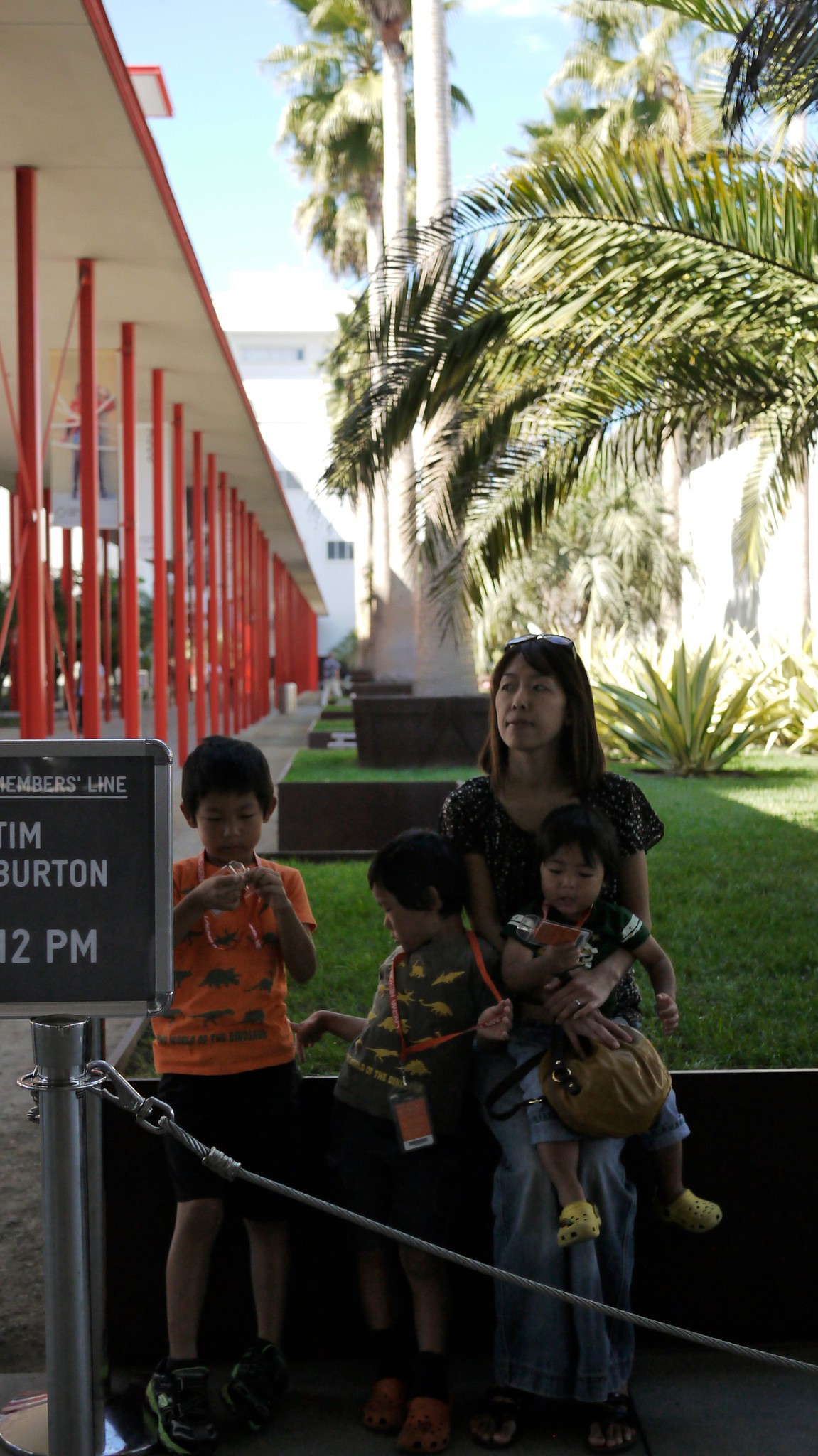The image depicts a woman standing outside with her three children, waiting in line for an event. The woman, who has short brown hair and is wearing a dark-colored short-sleeved shirt, rests against a half-wall. She has sunglasses perched on her head and is holding a young child in her left arm, who is wearing yellow crocs. To her left stand two young boys, one in an orange shirt and dark shorts. In front of them is a black sign with a silver frame that reads, "Members Line, Tim Burton, 2 p.m." The sign is accompanied by a black rope used to organize the queue. In the background, on the left, there is a row of red poles supporting a white roof of an open-air hallway, behind which are palm trees and a grassy area. The scene suggests they are waiting to attend a Tim Burton exhibit on what appears to be a pleasant day.